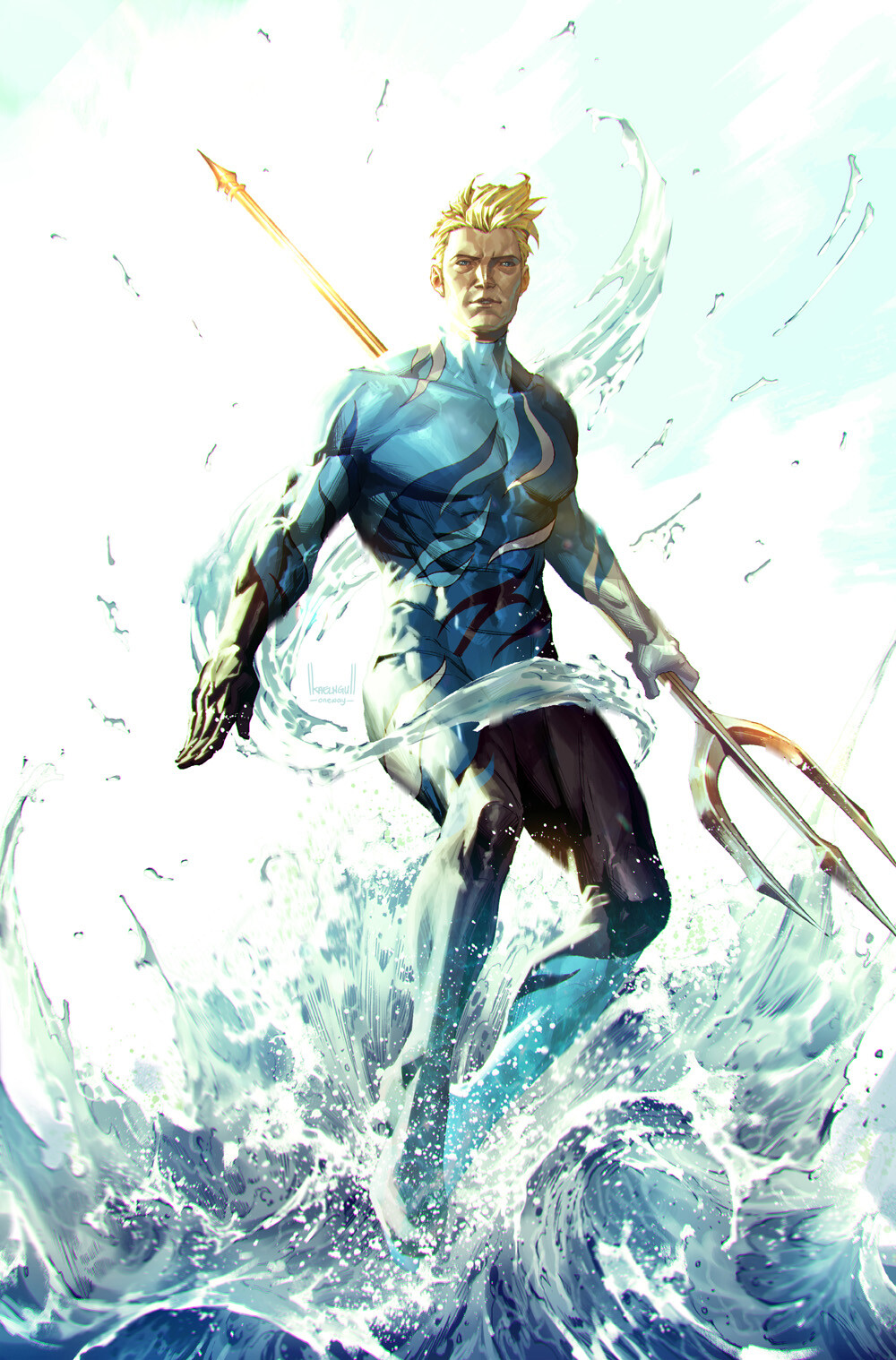The image is a detailed and animated comic book styled drawing of Aquaman, a DC superhero. It shows a muscular, white male with short, blonde, wavy hair and blue eyes, facing forward. Aquaman is clad in a tight, blue suit with black, white, and dark blue accents. His left hand grips a long, shiny golden and silver trident, which points downward. One glove is black while the other is silver, and he wears blue boots. The scene captures Aquaman rising out of a violently splashing pool of water, which swirls around him, creating dramatic waves filled with white foam. The sky above is a soft blue adorned with light clouds, enhancing the dynamic and heroic atmosphere of the image.